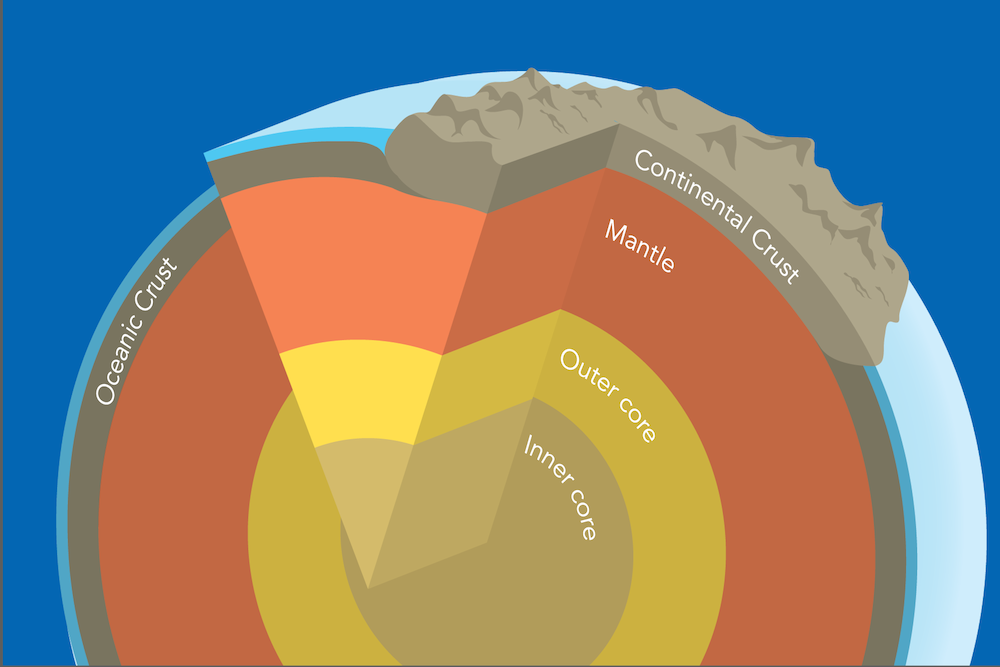The image is a detailed, colorful digital rendering of the Earth's internal layers, depicted in a simplistic, cartoon-like style. The illustration, set against a bright blue background, presents a cross-sectional view of the Earth with each layer distinctly colored. The outermost layer, representing the Earth's surface, is edged in a light blue indicating water or land boundaries. 

Starting from the outer edge, the light blue or turquoise layer signifies the Earth's surface. This transitions into the continental crust, illustrated with simplistic mountain shapes in grayish-brown, and the oceanic crust in a darker gray. Both types of crust contain textual labels. 

Below the crust lies the thick mantle, depicted in orange. Each deeper layer is meticulously labeled: the outer core in a deep yellow and the inner core at the very center, represented in a beige or khaki color. The background enhances the diagram's prominence, making the simplified, colorful depiction of Earth's layers stand out distinctly.